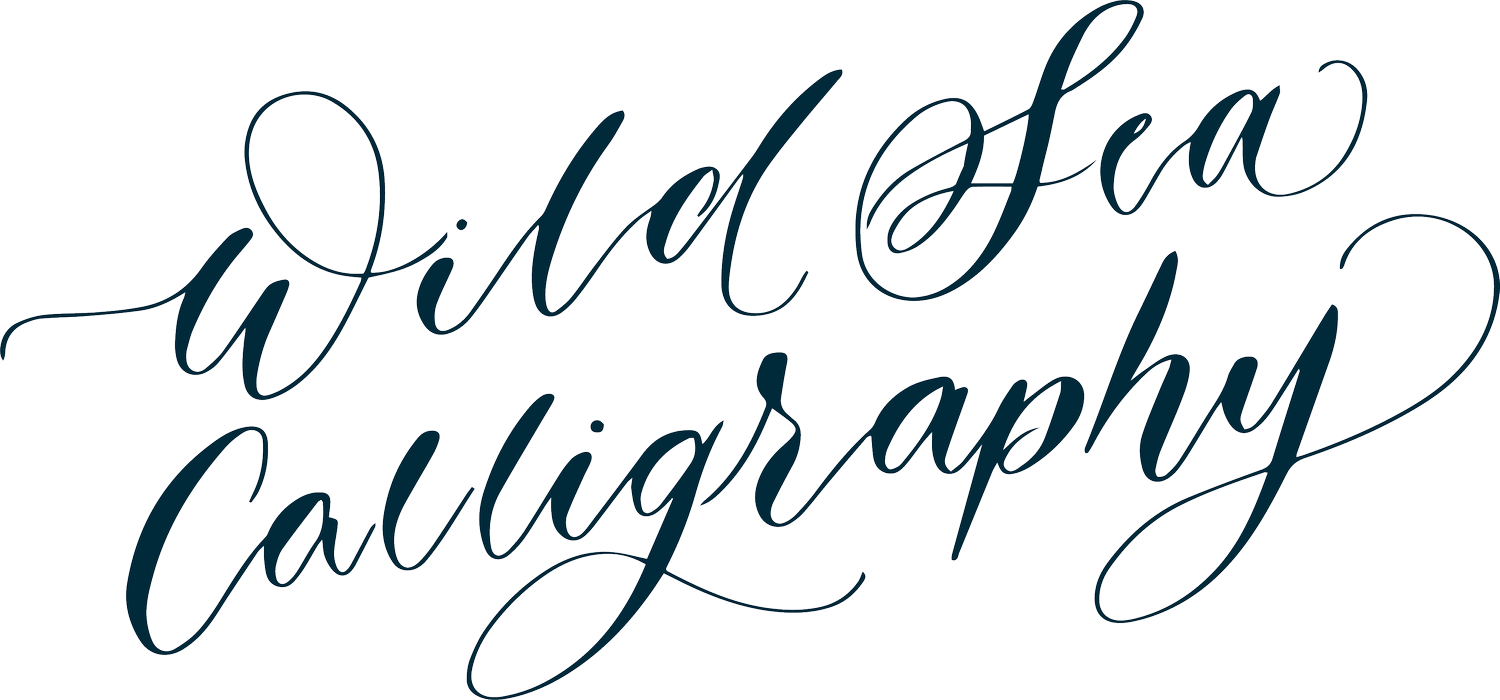The image features a decorative calligraphic text with no background, set against a plain, solid white backdrop. The text reads "Wild Sea Calligraphy" and is written in either black or dark blue ink. The calligraphy font is characterized by its cursive, right-top-to-bottom-left slant, with letters that have very slim, ornate endings, which are not simply curved lines but rather intricate, fancy loops. The design of the text shows varying weights, adding a visually striking contrast where some parts are darker and thicker, while others taper to fine, delicate lines.